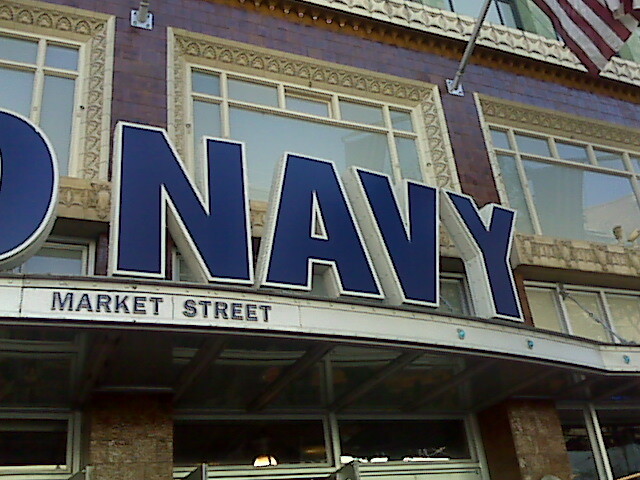This daytime color photograph showcases the storefront of a brick building on Market Street, prominently featuring an Old Navy store. The visible portion of the sign displays bold, blue, capital letters spelling "Navy," with the partial letter "D" from "Old" discernible. The storefront is executed in a detailed and sophisticated architectural style. The building features ornate window sills and sophisticated molding on the second story with large, rectangular plate glass windows, framed by smaller rectangular panes. The first story showcases plain, functional department store windows.

The sign sits atop a curved metal marquee with rivets, which projects outward above an open door area, suggesting a welcoming entry to the store. Under this marquee, the words "Market Street" are visible. Extending from the right side of the building, an American flag is seen, adding a touch of patriotic flair to the storefront. Another flag pole base is also discernible on the left side, though the flag it supports isn't fully visible. The intricate stone detailing and sophisticated appearance, combined with the marquee, give the storefront a unique visual appeal, distinctive from the more common mall or strip mall locations where Old Navy stores are typically found.